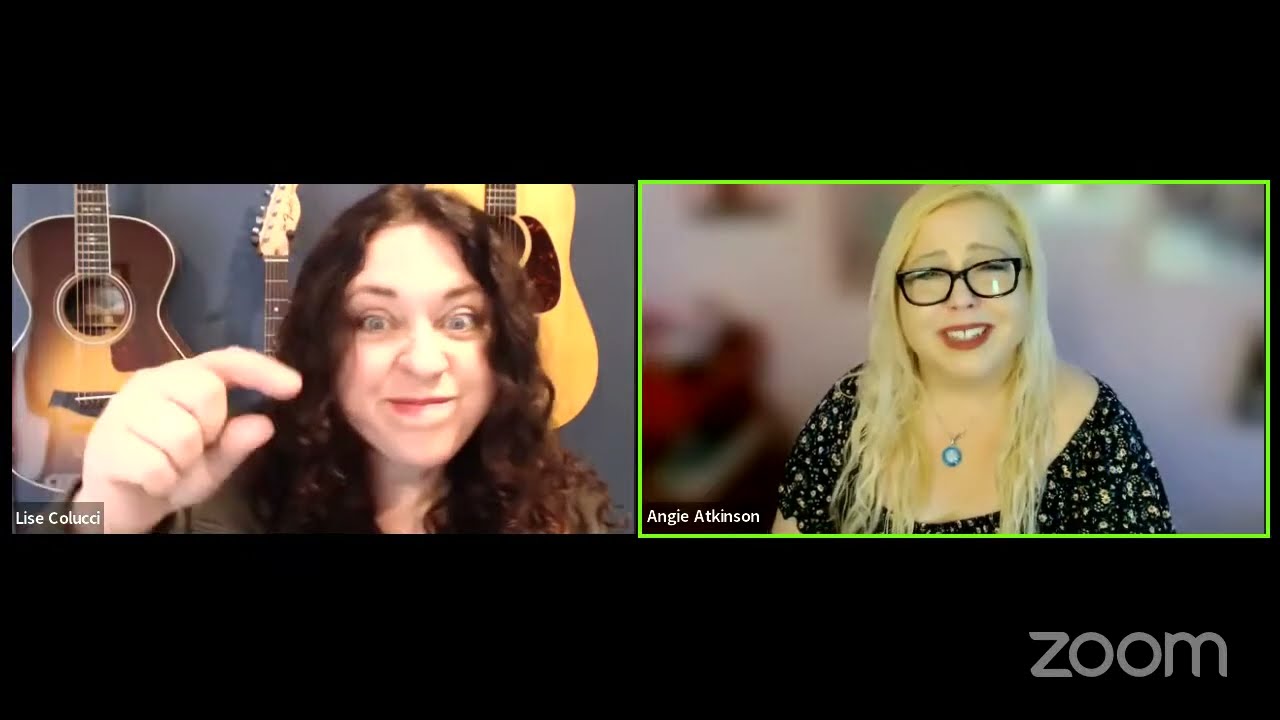The horizontal rectangular image is a screenshot of a Zoom meeting featuring two women in separate frames, bounded by thin black borders on the top and bottom. The right frame, outlined with a green box indicating the active speaker, shows a woman with shoulder-length blonde hair and black-rimmed glasses, wearing a black dress. She has a blue circular necklace and is seen with red lipstick. Her Zoom background is blurred. The left frame contains a woman with long dark hair, making a hand gesture with her right hand, where her index and thumb are extended while her other fingers are curled under. She has a humorous expression, seemingly making a joke, which is eliciting a laugh from the woman on the right. The background behind her displays three guitars hanging on the wall. While their names are partially visible, the woman on the left appears to be named Lyse Coexed, and the woman on the right, Angie Atkinson. The word "Zoom" is marked on the lower right of the black border.